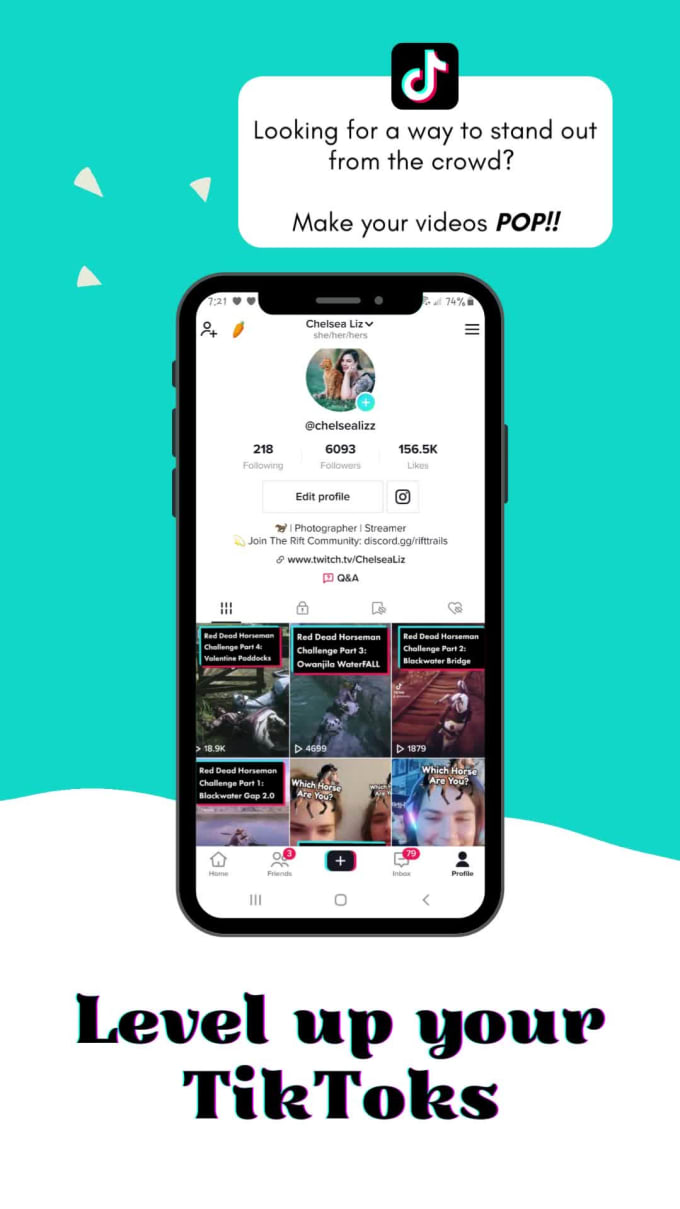The image features a teal-colored background with small, randomly scattered white triangular shapes concentrated on the left side. The bottom portion of the image transitions to white, where the text "Level up your TikTok" is prominently displayed in black letters. In the top right corner, the TikTok icon is placed above a white rectangle containing promotional text that reads, "Looking for a way to stand out from the crowd? Make your videos pop."

At the center of the image is a black smartphone displaying a TikTok profile. The profile header has a white background with the name "Chelsea" (though the text is very small and a bit unclear). Below the header, the profile showcases various metrics including followers and likes. Further down, six of Chelsea's videos are displayed in two rows of three, providing a snapshot of her TikTok content.